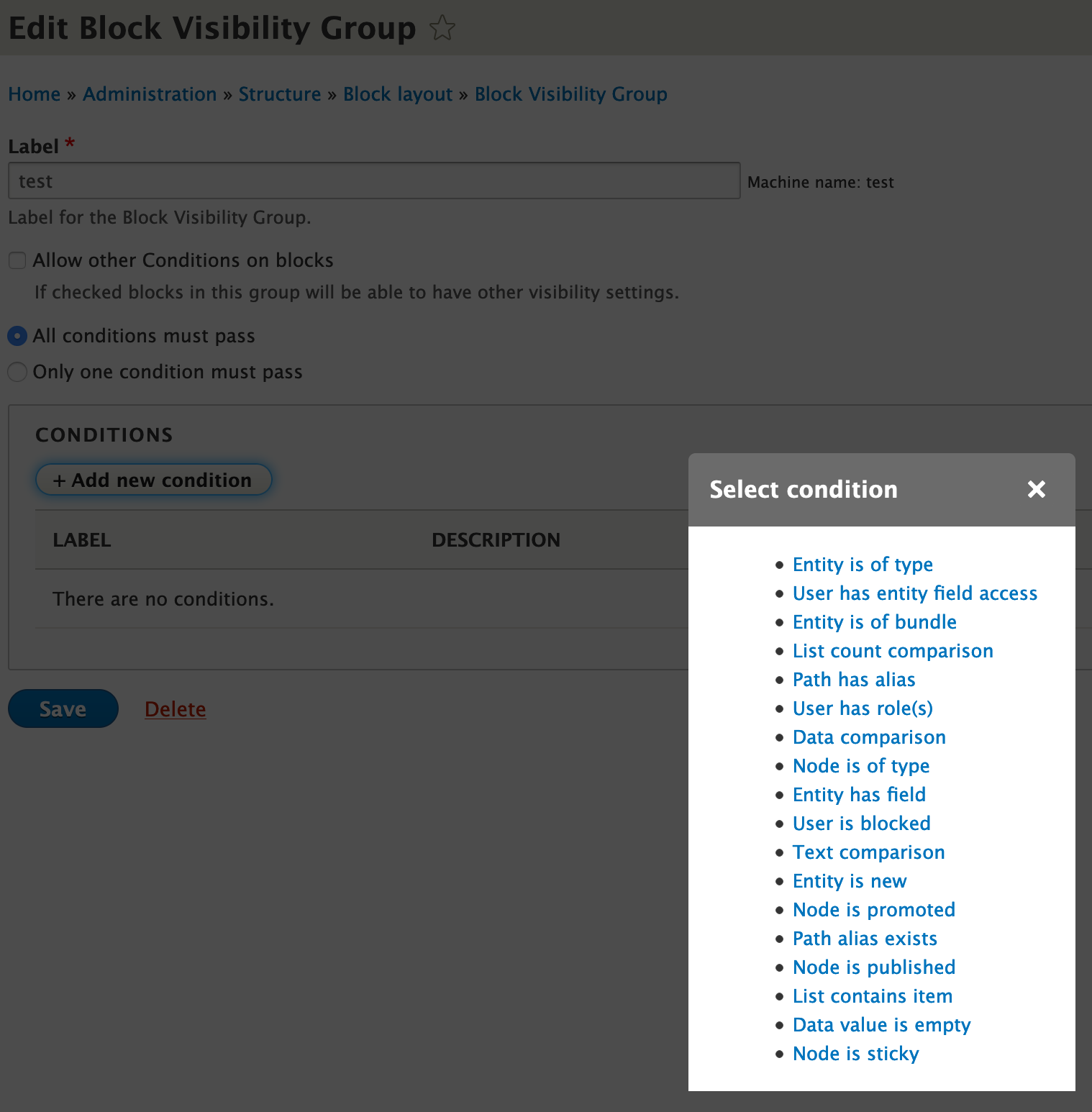The image depicts a web page obscured by a semi-transparent dark overlay, indicating the presence of an active pop-up window. The primary header of the page prominently displays the text "Edit Block Visibility Group." Below this header, there is a navigation menu with blue tabs arranged from left to right, labeled as: Home, Administration, Structure, Block Layout, and Block Visibility Group.

Within the pop-up window, the label "Label" followed by a mandatory field indicator (*) is visible. A text input box contains the word "Test," and at the right end of this box, it is labeled "Machine Name: Test." Beneath this, an explanatory line reads "Label for the Block Visibility Group."

Further down, there is an unchecked checkbox labeled "Allow Other Conditions on Blocks," followed by a description that states, "If checked, blocks in this group will be able to have other visibility settings." Below this description sits another checkbox, which is checked, labeled "All Conditions Must Pass," followed by an option "Only One Condition Must Pass."

The next section, titled "Conditions," features a clickable bubble with a plus sign labeled "Add New Condition," alongside fields labeled "Label" and "Description." Below these fields, the text reads "No Conditions" indicating that no conditions have been set.

Additional options presented include buttons to "Save" or "Delete" the configuration. The screen also displays a modal titled "Select Condition" featuring multiple bullet points with various options for conditions, such as: 
- Entity is of Type
- User has Entity Field Access
- Entity is a Bundle
- List Count Comparison
- Path as Alias
- User has Role or Roles
- Data Comparison
- Node of Type
- Entity has Field
- User is Blocked
- Text Comparison
- Entity is New
- Node is Promoted
- Path Alias Exists
- Node is Published
- List Contains Items
- Data Value is Empty
- Node is Sticky